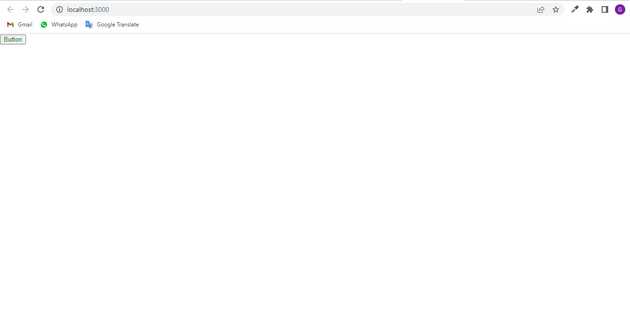A screenshot of a web page displaying a seemingly blank white canvas, possibly indicating an error or placeholder page, with an address bar showing "localhost:3000." This suggests it's a local development server, typically used by web developers for testing. In the top left corner of the page is a small, unstyled button labeled "button" in plain black text on a gray-green background. This minimal design implies it might be part of a test or prototype by a web designer, possibly a student experimenting with different techniques. Above the browser window, three bookmarked pages are visible: Gmail, WhatsApp (or a similar application), and Google Translate, hinting at the user's frequently accessed tools.